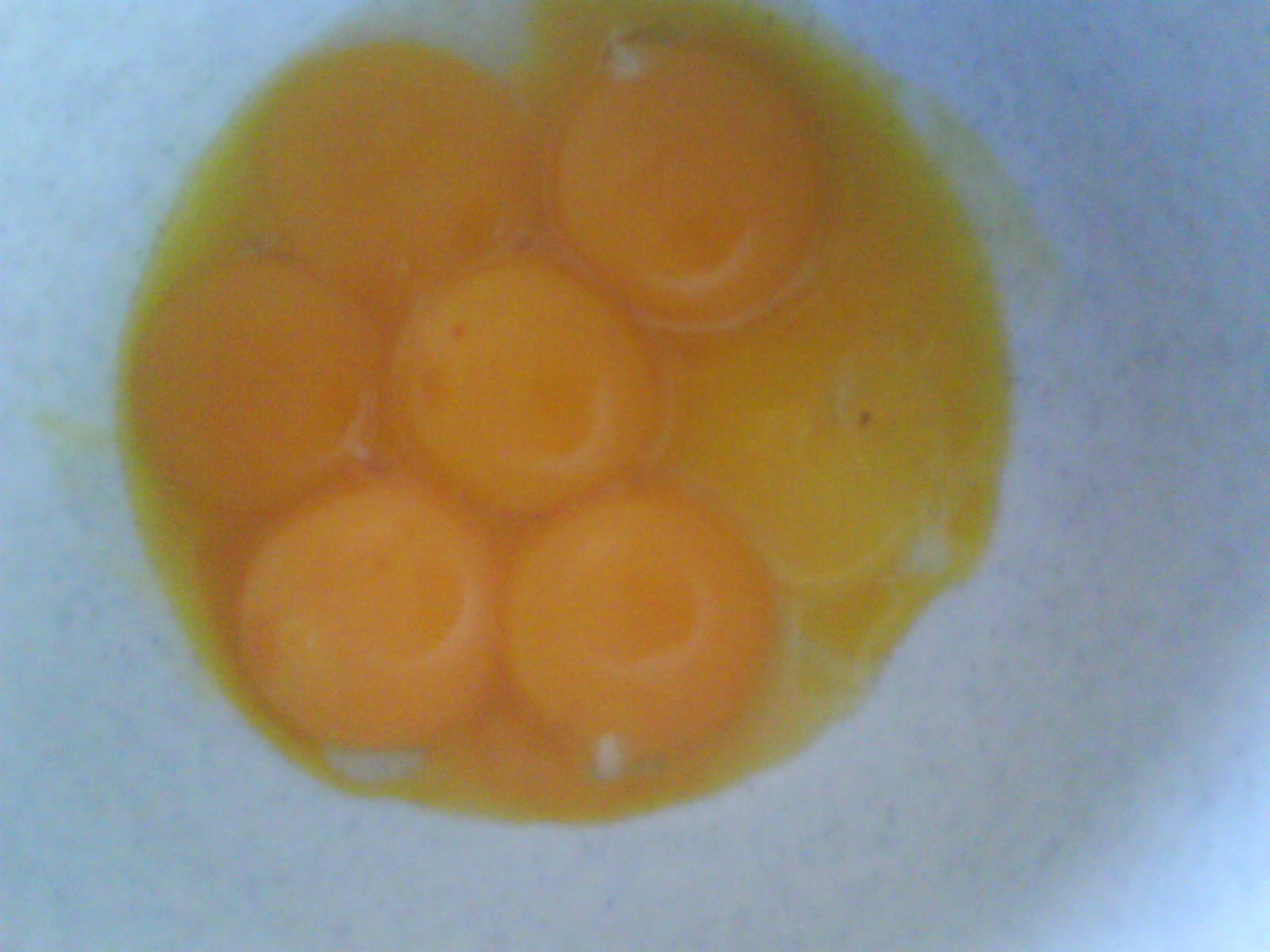This is a close-up, low-quality, blurry photo of six bright yellow and orangish egg yolks arranged in a roughly circular, flower-like pattern inside a light blue container. The yolks appear mostly intact with a visible spreading puddle and one broken yolk near the right side, around the three o'clock position. Small white specks, likely remnants of the albumen, are noticeable on a few of the yolks. The background, which seems indeterminate due to the blur, contrasts sharply with the vibrant yolks, making the composition more striking.